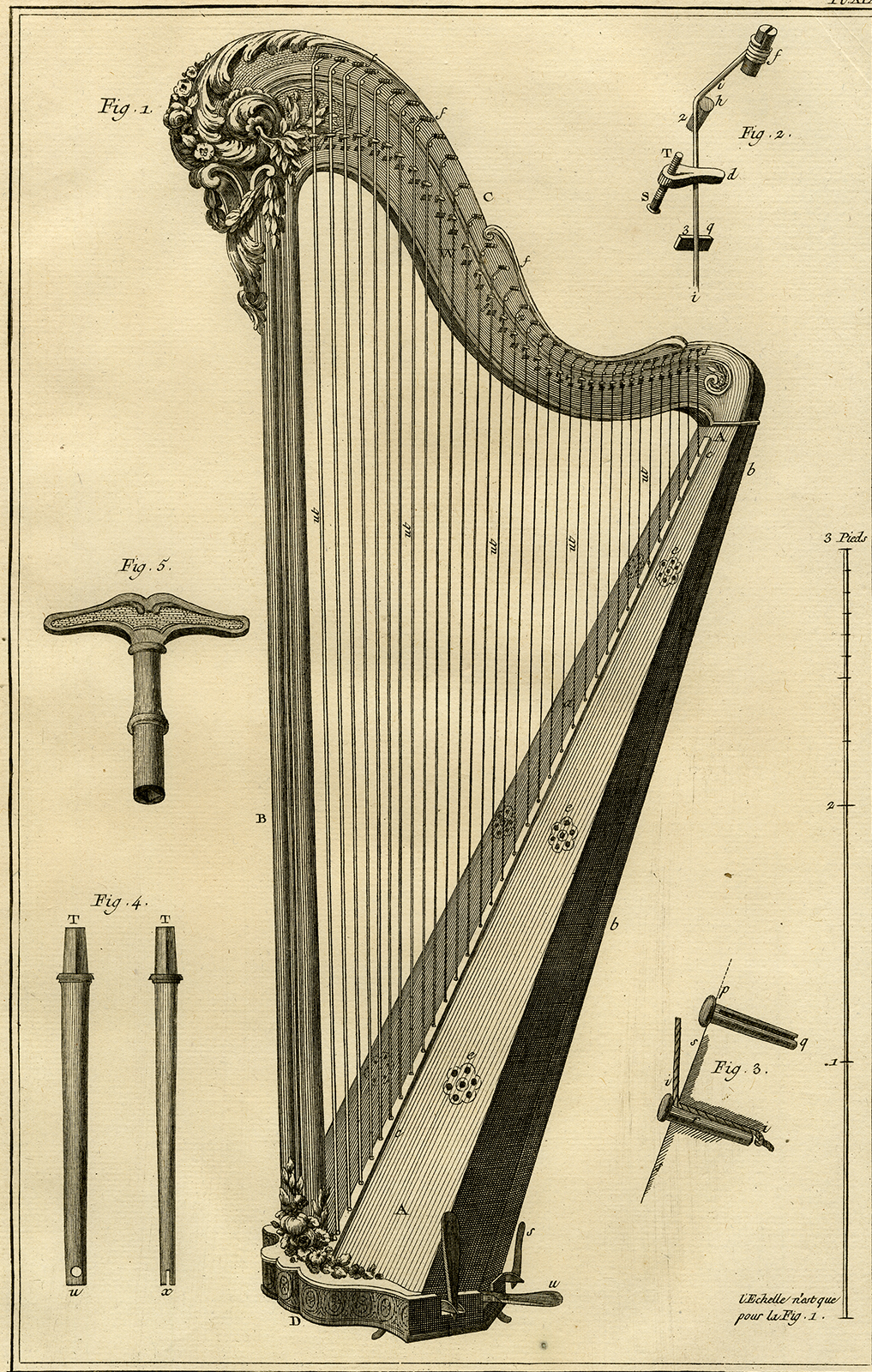This intricate poster features a highly detailed hand-drawn sketch of a harp and its various mechanisms, rendered in black ink on an off-white background with a subtle gray-green or pinkish hue. The central figure of the sketch, labeled Figure 1, is an ornate harp with a brocade-style floral pattern at the top, which gracefully flows down its curved neck. The harp's numerous strings and sculpted details are meticulously illustrated and labeled, capturing the instrument's elegance and complexity. Accompanying the main figure are several smaller diagrams: Figure 2 shows some string attachments, Figure 3 and Figure 4 depict long pegs possibly used for tuning, and Figure 5 illustrates a tuning key and an additional peg with spokes. Each element is annotated with numbers or letters, offering a comprehensive breakdown of the harp's components. This poster serves not only as a visual delight but also as an informative guide to the intricate parts of a traditional harp.